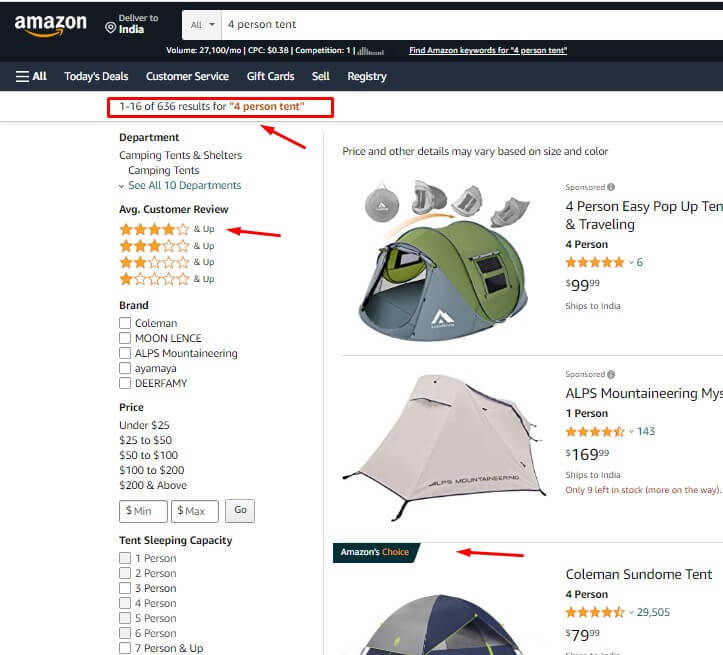The image depicts an Amazon search results page for the query "4 person tent." At the top, a dark banner reads "Amazon" with the delivery location set to India. Below this banner, there is a white search box labeled "4 person tent," accompanied by a dropdown menu option labeled "All." Underneath the search box, additional information is presented in white text, detailing the search volume as "27,100 per month," the cost-per-click (CPC) as "$0.38," and the competition level as "1." The text also promotes a keyword tool with the phrase "find Amazon keywords for 4 person tent."

Further down the page, there are header options such as "All," "Today's Deals," "Customer Service," "Gift Cards," "Sell," and "Registry." A red box with a red arrow highlights the text "1-16 of 636 results for 4 person tent."

To the right, several product listings are visible. The first product is a green "4 Person Easy Pop Up Tent for Traveling," boasting 5 stars from 6 reviews. The second product is a grey ALPS Mountaineering 1 Person Tent priced at $169. The last visible tent is the "Coleman Sun Dome Tent" in blue and grey, marked as "Amazon's Choice" with a red arrow pointing to it.

To the left of the product listings, navigation filters are provided. These include departments like "Camping Tents and Shelters," "Camping Tents," and an option to "See All Tent Departments." The filters also cover customer reviews, highlighted by a red arrow pointing to "4 stars and up," along with additional options for "3," "2," and "1 star and up." Further navigation options include selections based on "Brand," "Price," and "Tent Sleeping Capacity."